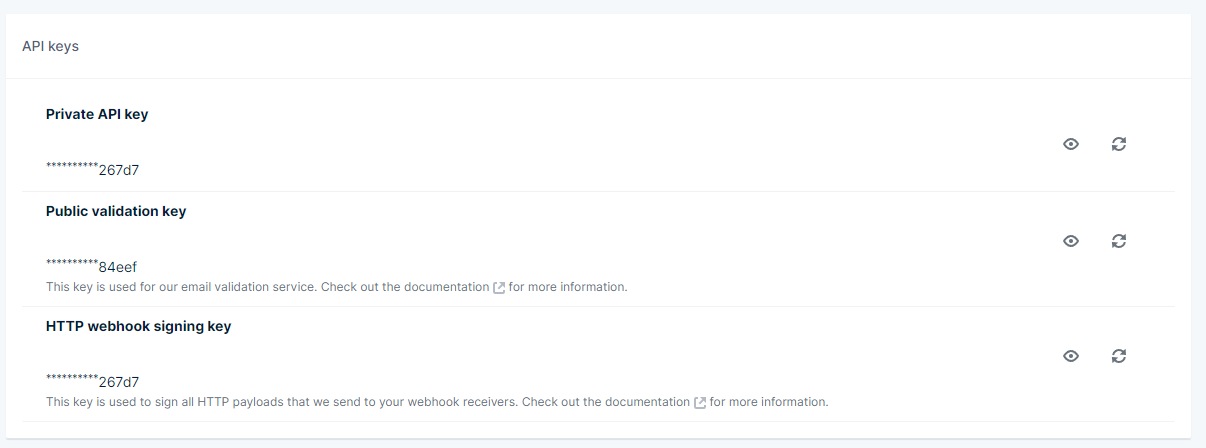The image portrays a webpage with a clean white background, detailing various API keys and their functionalities. 

1. **Private API Key**:
   - The section title reads "Private API Key".
   - The key itself is obscured with a series of dots, except for the last five characters, which are "267D7".
   - Two icons are present next to the key: one in the shape of an eye (presumably to toggle the visibility of the key) and another with a refresh symbol (presumably to generate a new key).

2. **Public Validation Key**:
   - The section title reads "Public Validation Key".
   - Similar to the private key, this key is largely obscured with dots, revealing only the last five characters, "84EEF".
   - This section includes the same two icons: an eye icon and a refresh symbol.
   - Below the key, in gray text, it explains: "This key is used for our email validation service. Check out the documentation for more information."

3. **HTTP Webhook Signing Key**:
   - The section title reads "HTTP Webhook Signing Key".
   - The key is again mostly hidden with dots, with the visible part being "267D7".
   - Icons for toggling visibility (eye icon) and updating the key (refresh symbol) are included, like in the other sections.
   - Below this key, gray text notes: "This key is used to sign all HTTP payloads that we send to your webhook receivers. Check out the documentation for more information."

The entire content is presented uniformly against a simple white background, emphasizing ease of reading and clarity.